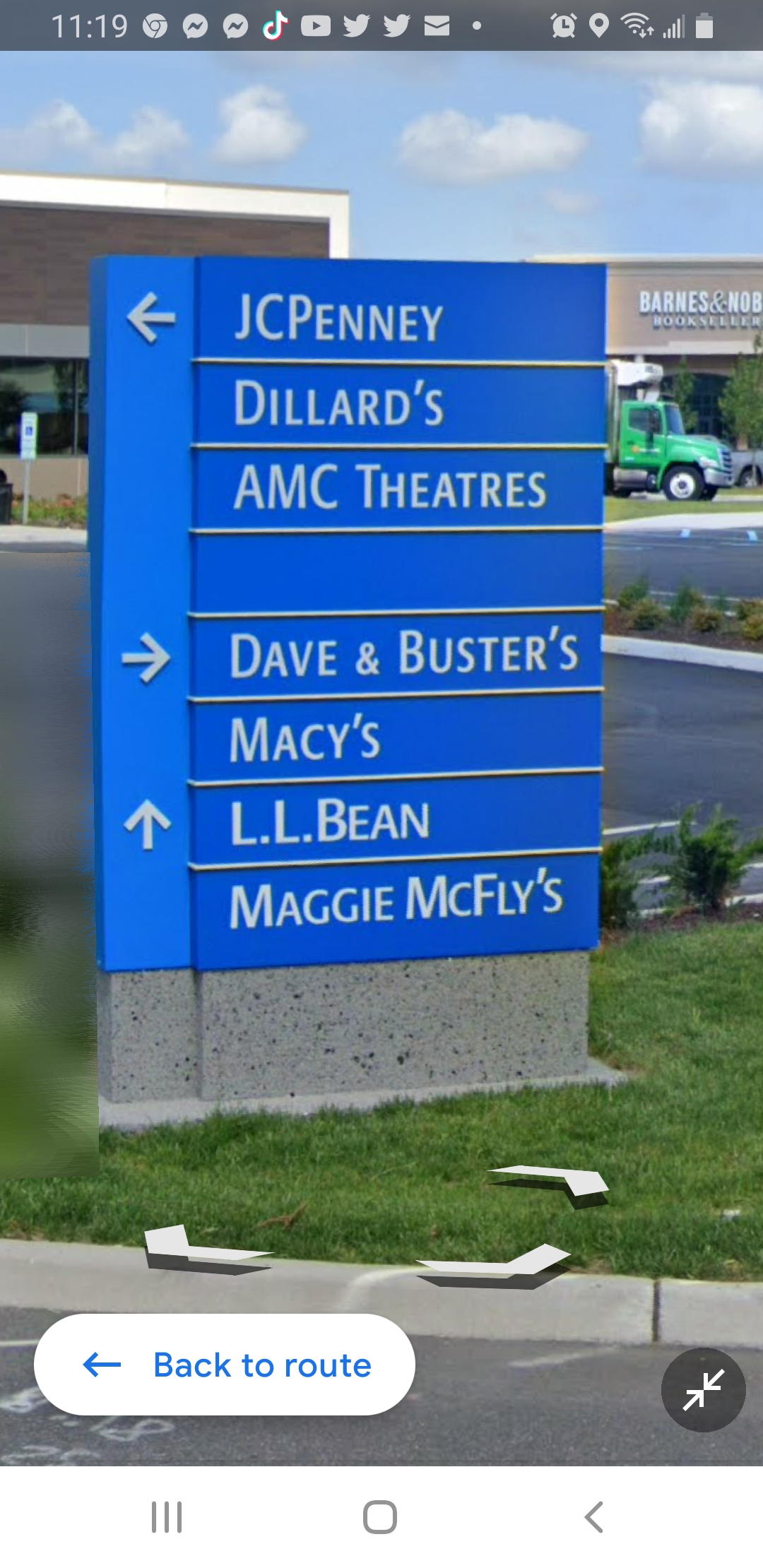This detailed image depicts a screenshot from an Android phone, capturing a vertical street view from Google Maps. Dominating the scene is a bright blue mall directory sign, mounted on a stone base, with distinct white text. The sign features arrows directing visitors to various popular stores and attractions: JCPenney, Dillard's, and AMC Theatres to the left; Dave & Buster's and Macy's to the right; and straight ahead to L.L. Bean and Maggie McFly's. 

In the background, there's a hint of a parking lot featuring a bright green truck, beyond which lies the recognizable storefront of Barnes & Noble. Another unidentified building is visible on the left side of the photo. Overlaying the image are several smartphone interface elements: at the top, there's a notification bar filled with alerts from apps like Messenger, TikTok, YouTube, Twitter, and Google Chrome, along with the time, noted as 11:19. At the bottom, typical Android navigation icons are visible, along with a white oval button labeled "Back to Route," likely part of the Google Maps interface.